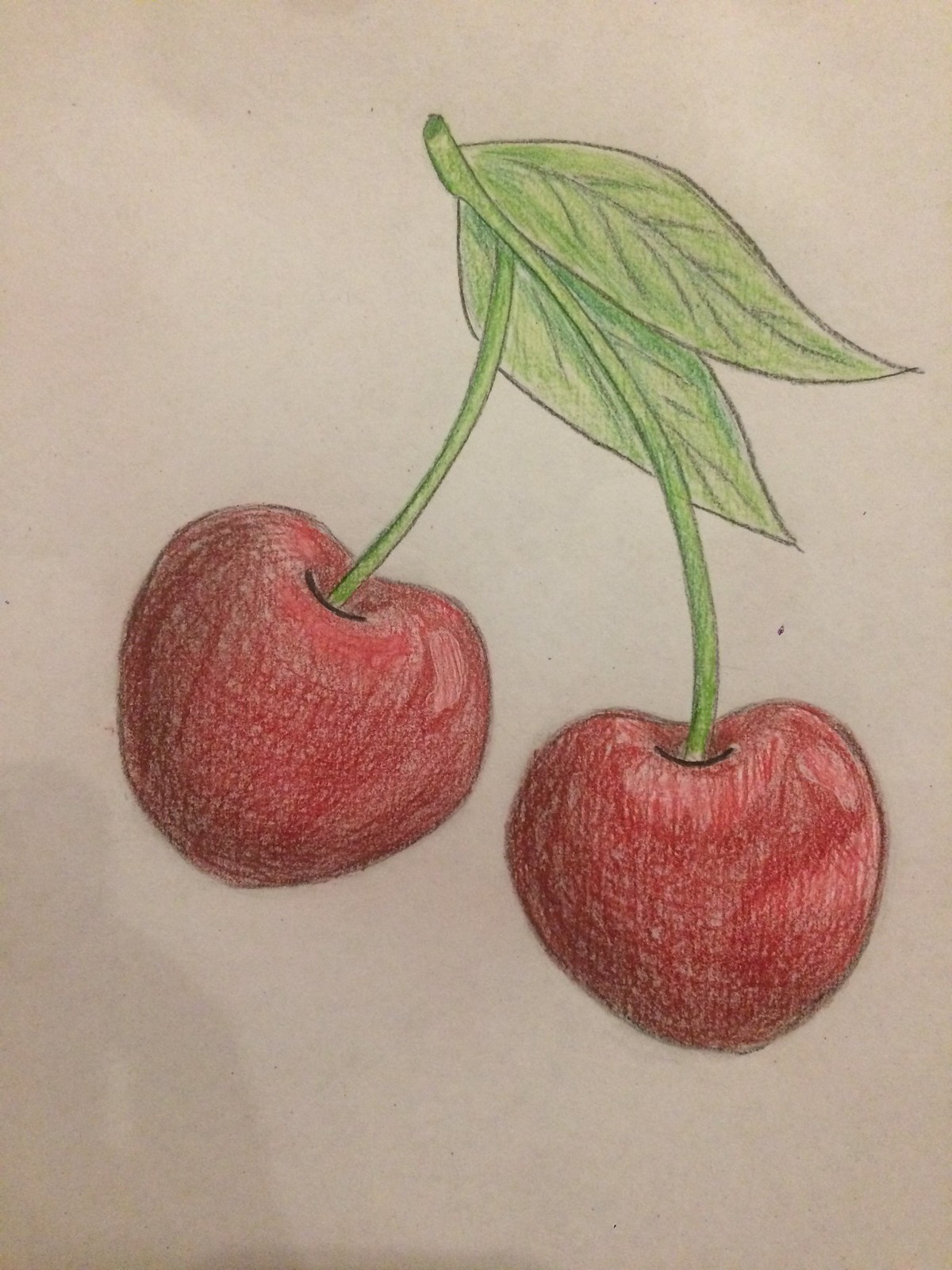The image depicts an artistic sketch of two cherries connected by their green stems and leaves, set against an off-white or light gray paper background. The cherries, reminiscent of the ones from Pac-Man, are colored with red pencils and detailed with white shading to illustrate their reflective surfaces. The stems intertwine and split towards the top, supporting two green leaves aligned with the right stem's curve. Each leaf showcases detailed vein lines drawn with darker pencils, giving a lifelike texture. The cherries feature subtle dark curves at the points where the stems attach, emphasizing depth. The shadows or possible stains on the bottom left corner suggest the picture was taken under varying light conditions.